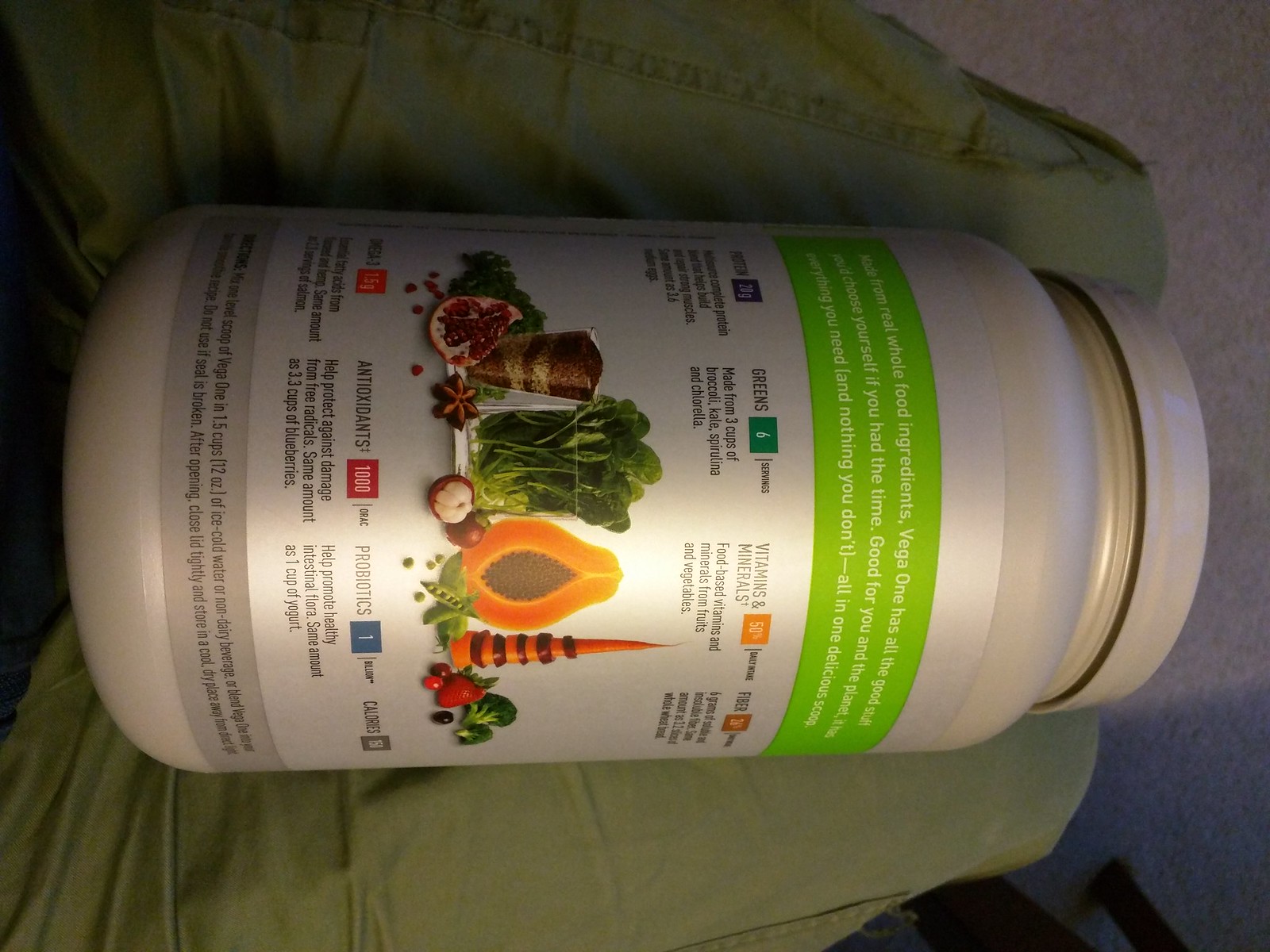In this image, the background features a neutral gray color, accompanied by a black chair partially visible. A light gray rug rests on the floor, adding texture to the scene. In the foreground, someone is wearing beige-colored pants, standing alongside a large white jug. The jug, capped with a white screw-on lid, prominently displays a green label encircling its middle. The label is adorned with colorful illustrations of various fruits and vegetables, including broccoli, carrots, and small tomatoes, suggesting the container holds a dietary supplement. The detailed imagery on the jug emphasizes a focus on healthy, nutritious ingredients.